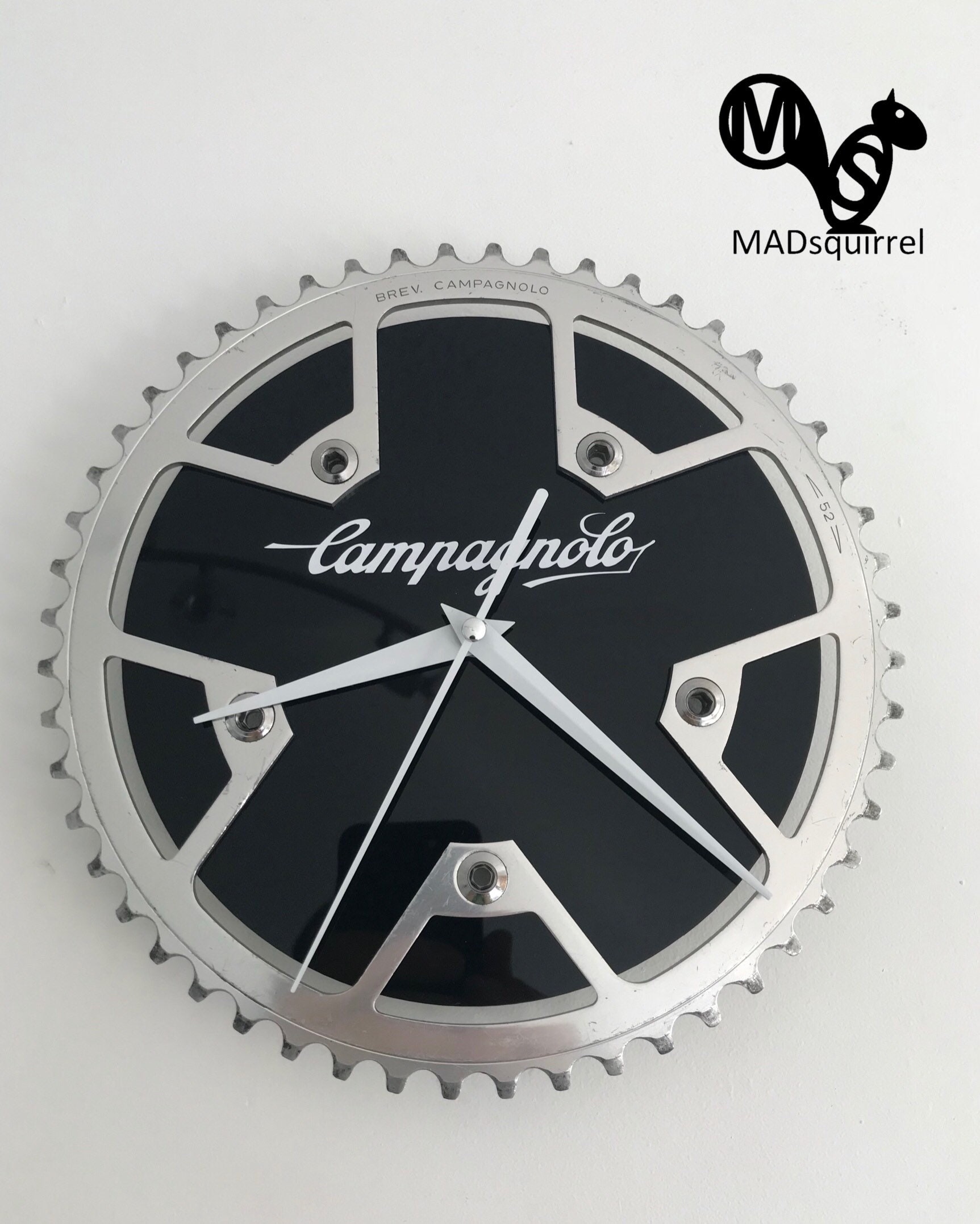This image features a unique clock creatively fashioned from a bike crank, prominently displaying the stylized logo of Mad Squirrel at the top right. The logo consists of a black squirrel design with the initials 'M' in its tail and 'S' in its body, along with a small white eye. Beneath this logo, the words "Mad Squirrel" are printed in black text. The clock itself is situated at the center of a metallic gear or cog, which serves as its outline. This gear has five trapezoidal protrusions, each equipped with screw holes or nuts, located at the 2, 4, 6, 8, and 10 o’clock positions.

The face of the clock is entirely black, free of any numbering, and features the cursive text "Campagnolo" at its center. Additionally, the upper part of the gear has the engraving "Breve Campagnolo" and the number "52" accompanied by thin arrows pointing left and right. The clock exhibits three metallic hands: a long minute hand extending to the gear’s edge, a shorter hour hand reaching about three-quarters of the way, and a slender second hand reminiscent of a chopstick that stretches to the perimeter of the gear. The clock shows the time at 9:20:35. The background of the entire image is white, enhancing the contrast and detail of the clock and logo.